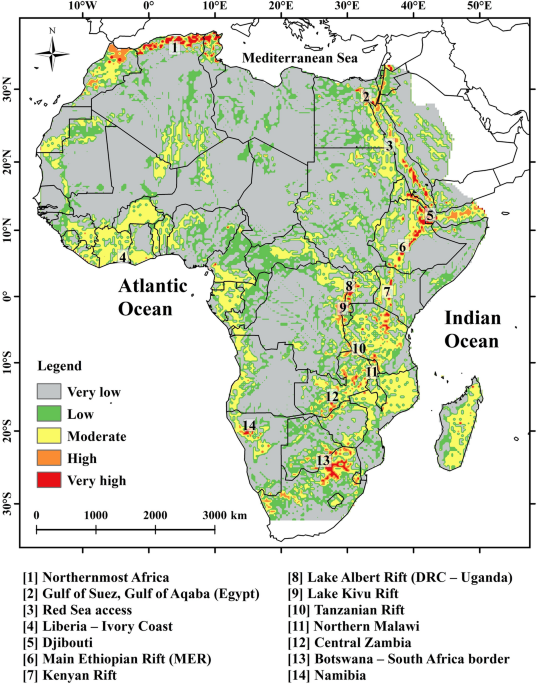The image is a detailed color illustration map of Africa with a portrait orientation. At the top of the map, the Mediterranean Sea is labeled, while the Atlantic Ocean is to the left and the Indian Ocean is to the right, positioned above Madagascar. The map features a white background with the African continent prominently outlined in gray, interspersed with patches of green, yellow, orange, and red, corresponding to a color-coded legend indicating varying levels: gray represents very low, green indicates low, yellow signifies moderate, orange stands for high, and red denotes very high.

Accompanying the map are two columns of black text numbered 1 through 14, which align with the colored patches on the map. These numbers correspond to specific regions or features within Africa, such as the Northernmost Africa, Gulf of Sousses, Gulf of Aqaba (Egypt), Red Sea access, Liberia, Ivory Coast, Djibouti, main Ethiopian rifts, Kenyan rifts, Lake Albert rifts (DRC, Uganda), Lake Kivu rifts, Tanzanian rifts, Northern Malawi, Central Zambia, Botswana-South Africa border, and Namibia. 

The map also includes notations of latitude and longitude along its top edge and left margin. A compass is placed in the top left corner, and below the map, a legend explains the color-coded elevation or other criteria, with a scale of inches and kilometers assisting in distance measurement. Despite the detailed representation, the map's purpose or what the levels specifically stand for is not explicitly stated.